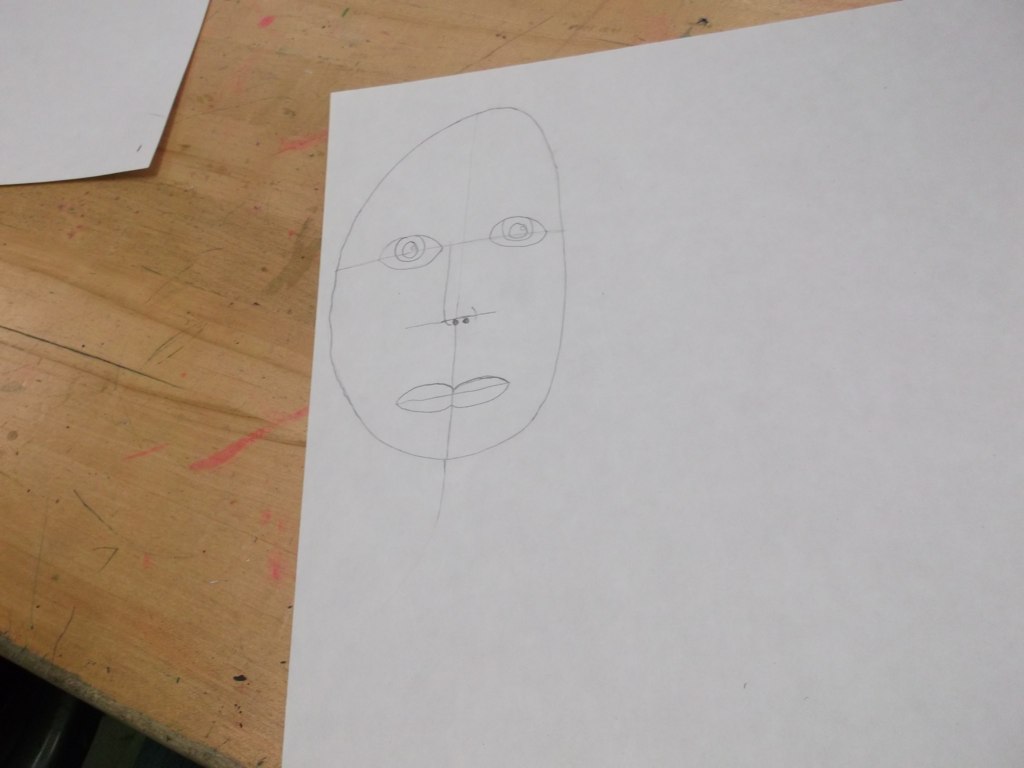This image showcases a detailed drawing on a white piece of paper, lying on a worn, scratched desk with noticeable red marker stains. In the upper left of the drawing, there is a meticulously sketched oval face. The face is drawn with striking symmetry, highlighted by guidelines that intersect at the center; one vertical line runs from the top to the bottom of the oval, and one horizontal line spans across the middle. These guidelines align the facial features precisely. The eyes, positioned along the horizontal line, are detailed with distinct pupils. Below, a thin nose is carefully rendered, leading down to well-defined lips. In the upper left corner of the image, another sheet of paper is partially visible, contributing to the scene.